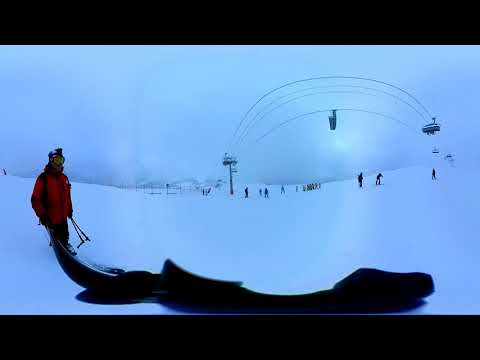A skier dressed in a red jacket, possibly with matching red or dark pants, stands on the left side of the image. He is wearing wide plastic goggles and a ski mask, holding ski poles in his left hand and dragging a long black object with his right. The photograph is taken using a fisheye lens, which distorts the scene, making straight lines appear curved. In the center of the image, ski lift cables curve dramatically due to this lens effect, with gondolas swinging underneath. The snowy ski slope stretches out beneath a thick, cloudy sky, with the sun barely piercing through the overcast conditions. The resort is populated but not crowded, with more than ten skiers spread across the slopes in the distance. The image feels misty and foggy, with some indistinct fence panels visible near the ski lift in the far distance. The combination of the skier's abstract shadow and the distorted perspective creates an unusually compelling visual.